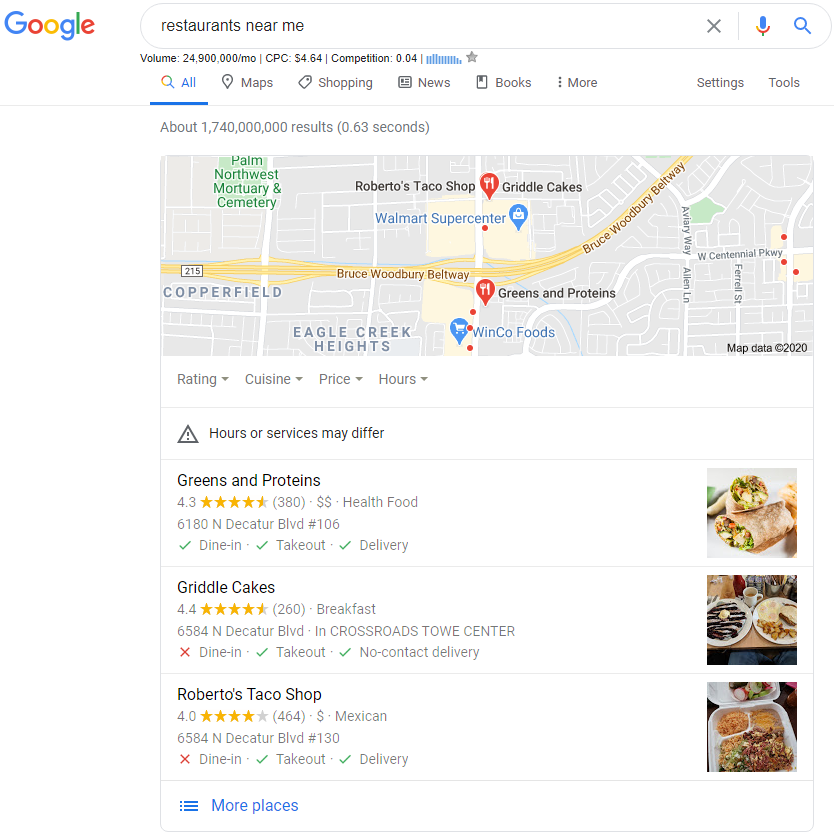A search is conducted on Google with the query "restaurants near me" displayed in the search bar. Below the bar, search metrics are presented: 24,900 in volume, CPC at 464, and competition rating at 0.04. The standard Google navigation options, such as "All," "Maps," "Shopping," "News," "Books," "More," "Settings," and "Tools," are available.

A map displays an area labeled Eagle Creek Heights, with a green marker indicating the Palm Northwest Mortuary and Cemetery. Beneath the map, there are options to filter restaurants by ratings, cuisine, price, and hours of operation, along with a note that "hours of service may differ."

Three restaurants are listed:
1. **Greens and Proteins** – Rated 4.3 stars, accompanied by an image of a burrito. 
2. **Griddlecakes** – Rated 4.4 stars, specializing in breakfast. Options include dine-in, takeout, and no-contact delivery. The image showcases pancakes.
3. **Roberto's Taco Shop** – Rated 4.0 stars, offering Mexican cuisine. Dining options include dine-in, takeout, and delivery, with an image depicting Mexican food in a takeout container.

At the bottom of the listings, a blue link labeled "More places" offers additional restaurant options.